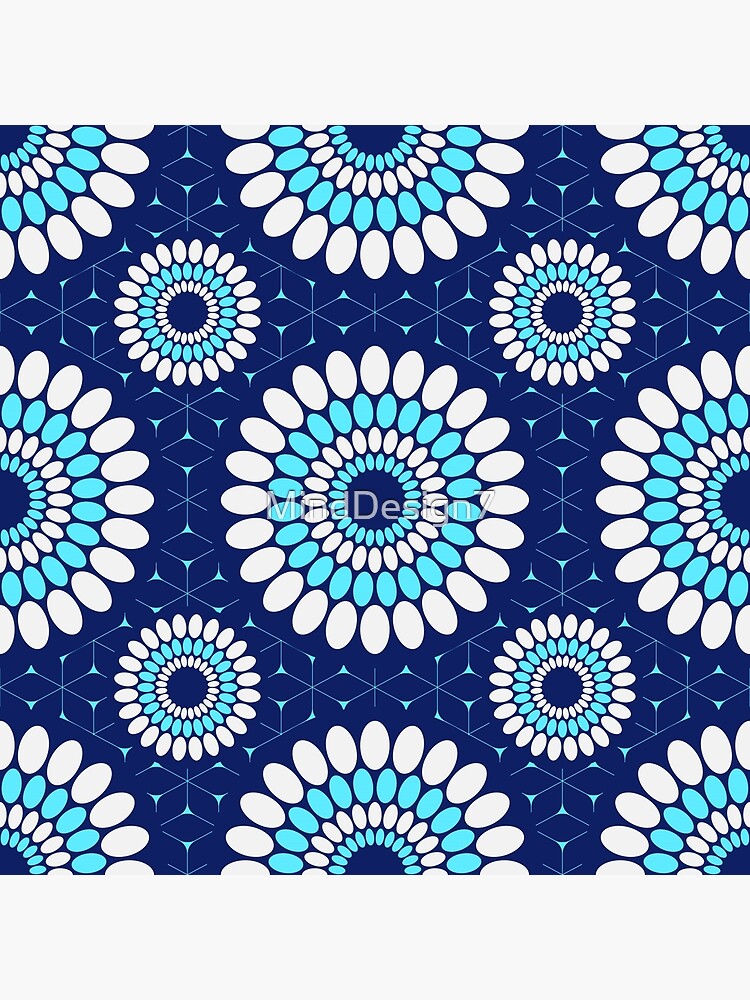The digital graphic presents a symmetrical design characterized by a repeating floral pattern set against a dark blue background. The background itself is accentuated with a light blue grid, forming squares that contrast with the primary dark blue shade. At the center, the graphic prominently features the text "Mine Design 7." 

The focal point of the design is a series of concentric circular patterns composed of ovals or egg-like shapes. These circles alternate between light blue and white, creating a visually striking effect. The innermost circle has a dark blue center, followed by layers of light blue, white, light blue, and white ovals. Surrounding the central large circle, smaller iterations of the same pattern are positioned at each corner—top right, top left, bottom left, and bottom right.

Additionally, colorful rose petal-like elements, with dark blue centers and concentric circular patterns, are scattered across the design, contributing to the wallpaper-like, repeating motif. The interstitial spaces between the ovals feature lines with triangles at their ends, forming X shapes that add another layer of geometric interest to the intricate design.